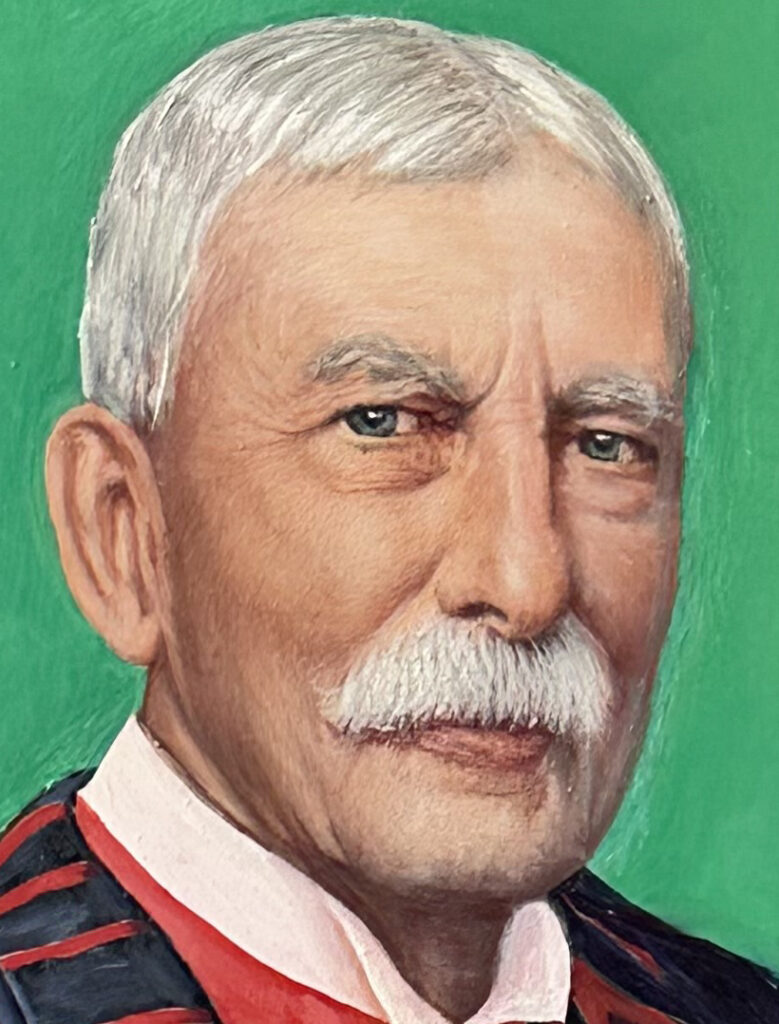The image is a detailed, realistic painting of an older man, likely between 65 to 70 years old, with white skin and neatly combed short gray hair, which appears almost white in some places. His blue eyes and bushy gray eyebrows frame his face, accented by a prominent white mustache that does not extend beyond his mouth. The portrait captures his head, neck, and just the tops of his shoulders, suggesting a close-up view. The man wears a white collared shirt, underneath a black jacket with red stripes. The background is a textured, spring green hue with visible lines from the paint or pencil, adding an additional layer of detail and authenticity to the artwork. The man is looking to the side, and his larger ears and regular-sized nose and mouth are clearly depicted, emphasizing his attentive demeanor.